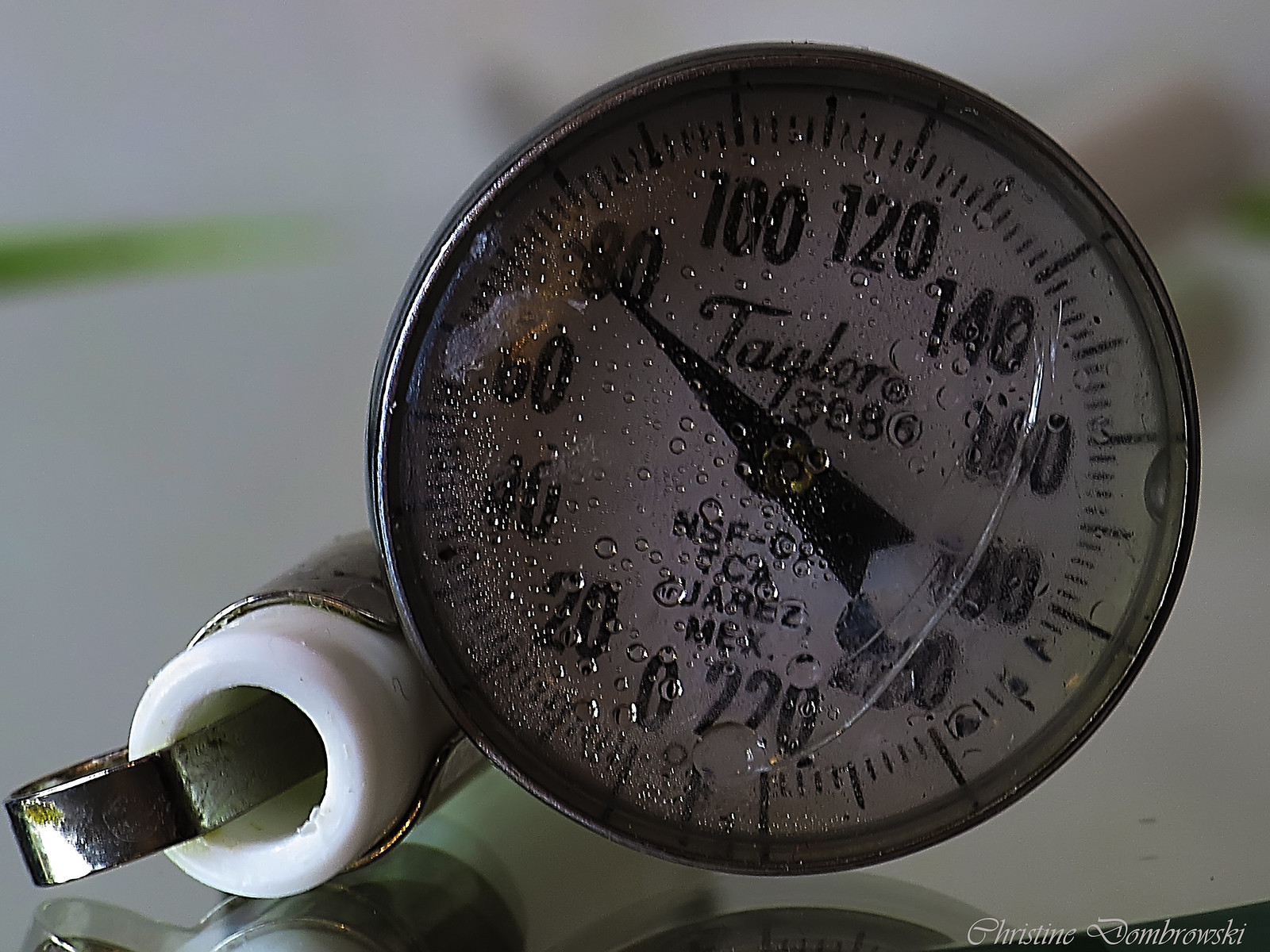The image features a prominent, slightly wet gauge in the foreground, displaying a scale from 0 to 220, marked with small dashes. The backdrop is blurred, suggesting a slightly chaotic setting. In the bottom right corner, a signature reading "Christine Zombrowski" is visible, likely indicating the author or artist. To the left of the gauge, a cylindrical object is noticeable, partially obscured by a white bottle. A silver instrument protrudes from this bottle, extending outward. Additionally, a fine crack runs across a section of the screen, adding to the image's textured and somewhat aged appearance.